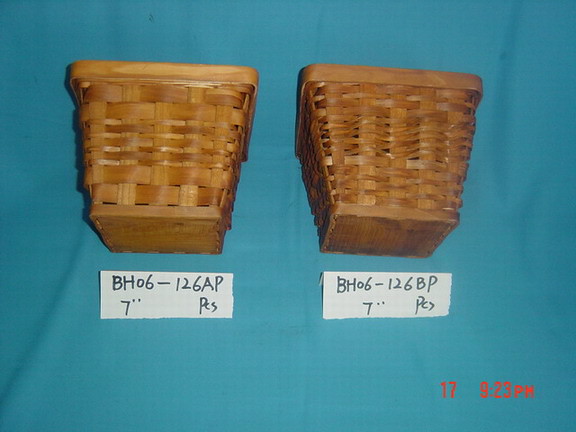In the photograph, two square, woven brown wicker baskets are prominently displayed against a blue fabric background. Each basket lies on its back, showcasing both its flat bottom and open top. The basket on the left features a flat piece of wood on its base and is slightly less tightly woven compared to its counterpart on the right. Each basket is labeled with a white piece of paper positioned underneath. The left label reads "BH06-126AP, 7 inches, PCS," while the right label reads "BH06-126BP, 7 inches, PCS." In the bottom right corner of the image, the red text "17 923PM" is clearly visible. Both baskets measure approximately 10 inches tall and 8 inches wide.